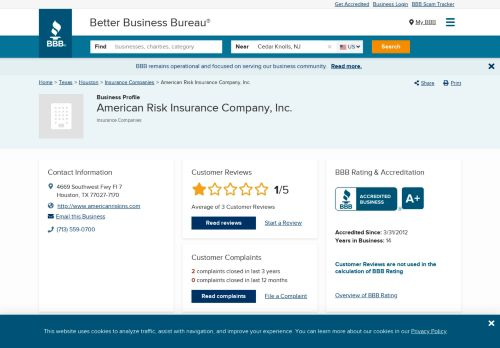The image is a screenshot of the Better Business Bureau's (BBB) business profile page for American Risk Insurance Company. In the top right corner, there's text reading, "Get appreciated, get credit. Business login." The name "Penn and Hemberman" appears, possibly authors or contributors. The business is located near Cedar Knolls, New Jersey, in the United States.

The webpage includes several yellow rectangular buttons for navigation, such as "Search", "Home", "Team", and "Insurance Companies." The business profile section prominently displays the name "American Risk Insurance Company" and provides options to "Share" and "Print" the page.

On the left, there's contact information:
- Address: 660 Southwest, Houston, Texas
- Website: [www.americansrisk.com](http://www.americansrisk.com)
- Email: [provided email]
- Phone: 713-556-9070

The customer reviews section indicates a rating of 1 out of 5 stars. It also mentions that there have been 2 customer complaints closed in the last year and 0 complaints closed in the previous year. Additionally, it notes 3 and 5 Bluebird complaints.

The BBB rating for American Risk Insurance Company is an A+, and it has been accredited since 2009 and 2012 respectively, with a business history of 36 years. The website also uses cookies for analysis purposes.

Overall, the image succinctly provides detailed information on the business's performance, consumer feedback, and contact details, offering a comprehensive view of the company's standing with the BBB.